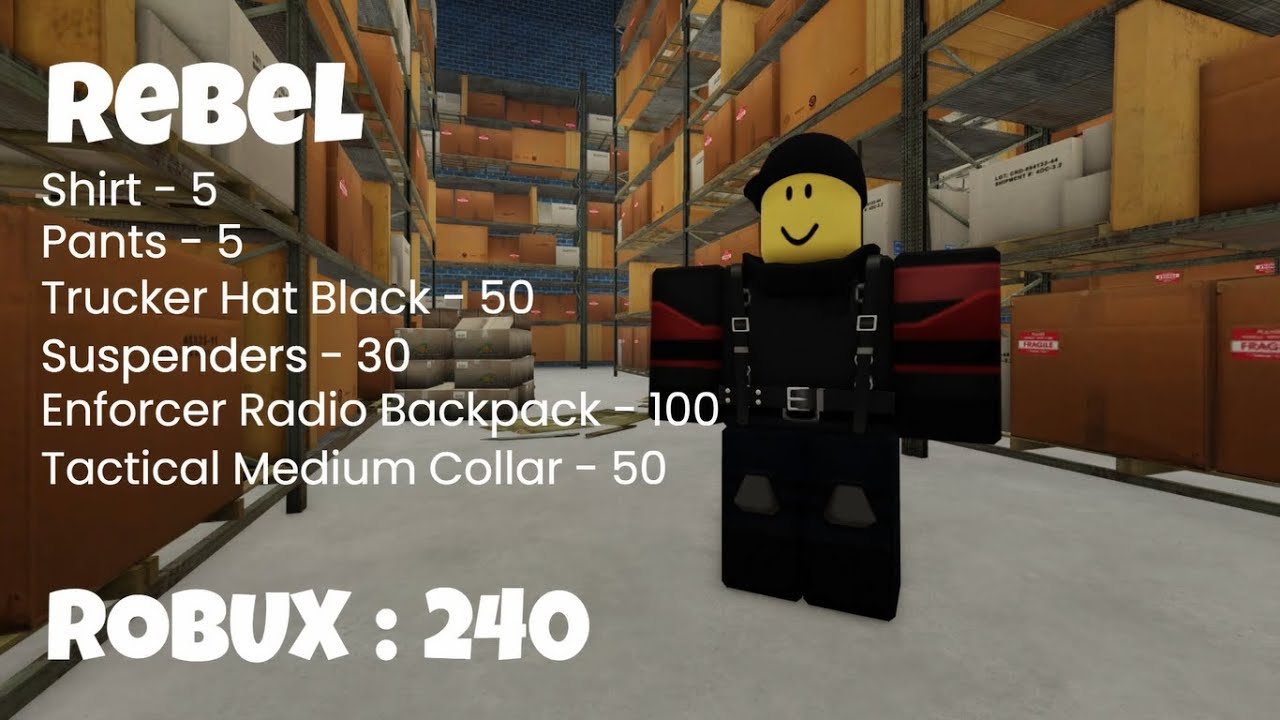The image depicts a 3D game-like environment set inside a shipping warehouse, characterized by tall shelving filled with brown and gray cardboard boxes, many of which are marked with red and white "fragile" stickers. The floor is a dark gray color, seen prominently at the center and bottom of the image. In the foreground, near the center, stands a 3D character resembling a Roblox figure with a yellow face, black cap, and black attire, including a jumpsuit and a harness featuring orange straps around its arms and a belt across its waist. The character exudes a happy demeanor with a smiling mouth. In the image's top left corner, the bold white text reads "REBEL," likely the character's name. Below this, additional details are listed in smaller, sans-serif white text: "SHIRT-5, PANTS-5, TRUCKER-HAT-BLACK-50, SUSPENDERS-30, ENFORCER-RADIO-BACKPACK-100, TACTICAL-MEDIUM-COLLAR-50." At the bottom, in large, bold white text, it reads "ROBUX-240," indicating the in-game currency value associated with the character.